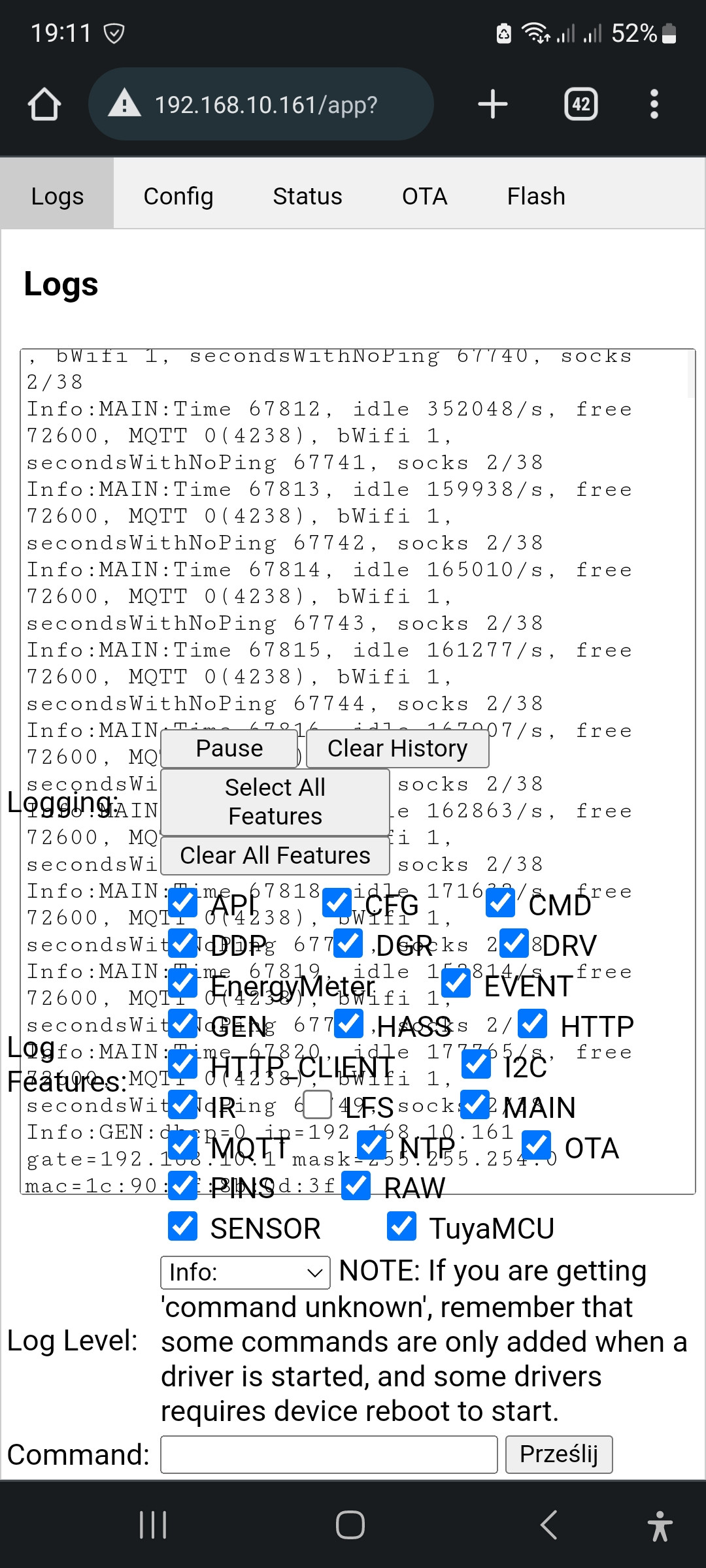This screenshot captures a mobile interface of a system or technical log page that appears to be slightly glitched. At the top of the page, there are several navigation tabs labeled "Logs," "Config," "Status," "OTA," and "Flash," with the "Logs" tab visibly highlighted. Below this, the main section displays detailed lines of data in a highly technical layout under the heading "Logs."

Further down, the interface includes options for adjusting the log level and inputting commands. Overlaying this information, a semi-transparent layer is visible that reads "Logging." This overlay obscures parts of the underlying technical data and includes buttons labeled "Pause" and "Clear History" for controlling the log display.

Additionally, there is a section with checkboxes allowing users to configure log features. These checkboxes are arranged in three columns, with the majority of them selected. However, due to the poor overlay alignment, the visibility of these checkboxes is impeded, making it challenging to discern their exact status.